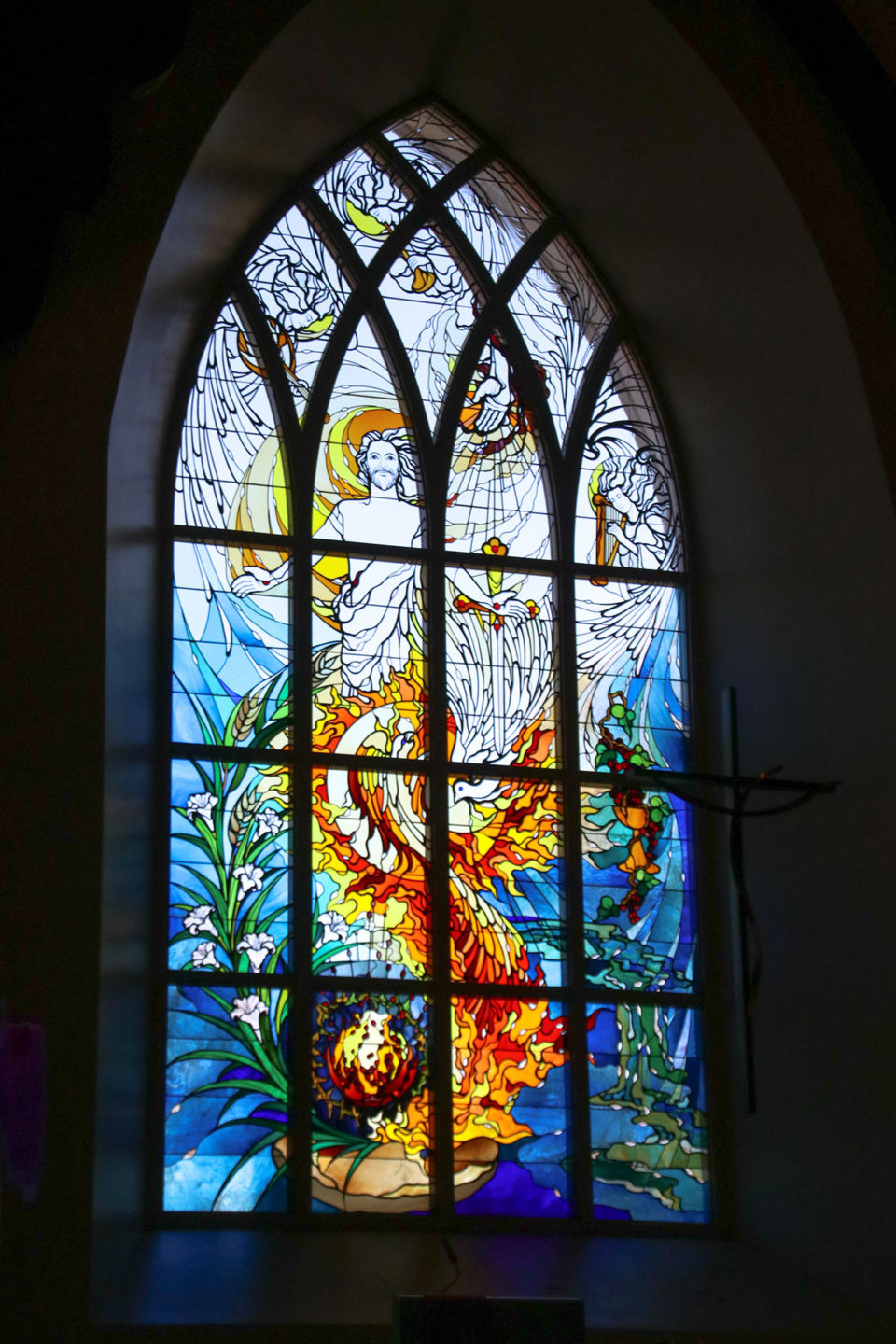This photograph captures an intricate stained glass window inside a building, illuminated by sunlight that highlights its vibrant colors. The window is designed with a 4x3 grid of squares topped by a 3-to-1 pyramid shape, moving from a pointed apex to parallel lines ending in a flat bottom. The scene depicted is rich and complex: in the center stands a figure that appears to be Jesus Christ, clad in traditional robes, holding a sword with his right hand, giving the impression of both guidance and sovereignty. Flanking Jesus are angels—some depicted playing harps—contributing to the celestial ambience. At the base of the window, vibrant flames swirl upwards, possibly from a campfire-like scene, entwining with what looks like a phoenix rising, symbolizing rebirth or transcendence. On either side of the flames, fluid-like blue areas evoke the imagery of water. Complementing these elements, various intricate details include a harp-playing figure to the right, a plant-like form reaching upwards from the bottom left, and hands descending from the top, possibly symbolizing divine interaction. The color palette transitions from sunset hues to serene blues and greens, executed in a beautiful Tiffany style, rendering it a visually and thematically rich masterpiece.